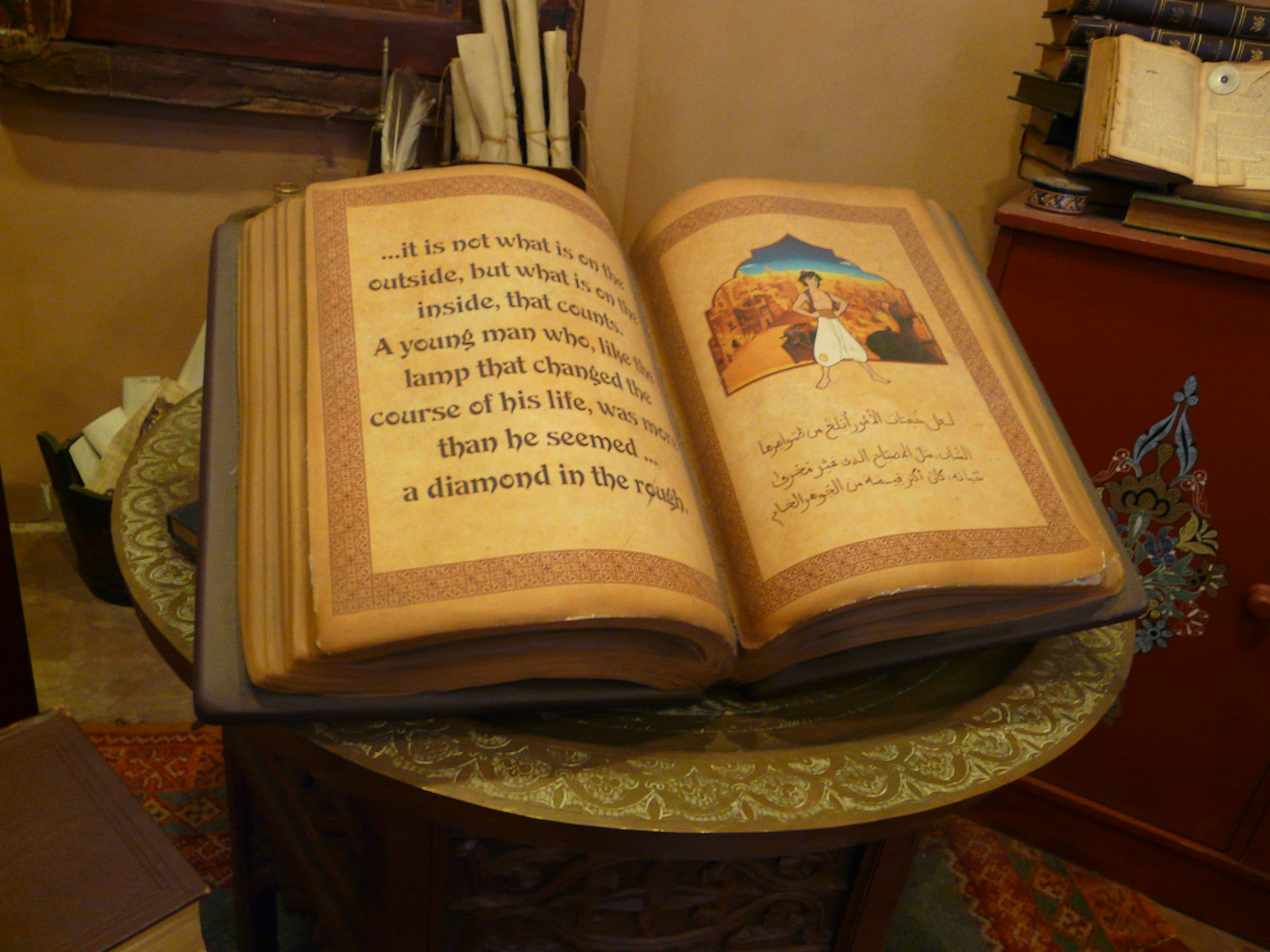The photograph showcases an indoor scene centered around an open book on a round wooden coffee table adorned with ornate golden details. The book, likely a prop due to its aged and yellowed pages, lies flat with a picture of Disney's Aladdin on the right page and Arabic writing underneath. The left page bears the text: "It is not what is on the outside but what is on the inside that counts. A young man who, like the lamp that changed the course of his life, was more than he seemed, a diamond in the rough." This setup, evocative of a Middle Eastern aesthetic possibly from the 1970s, is set against a background of tan, worn walls. To the right, a red dresser holds more books, some of which are open or stacked sideways. Additional details include a Persian rug beneath the table, and a container holding rolled pieces of paper. Another container nearby holds feathers, adding to the eclectic, vintage atmosphere of the scene.